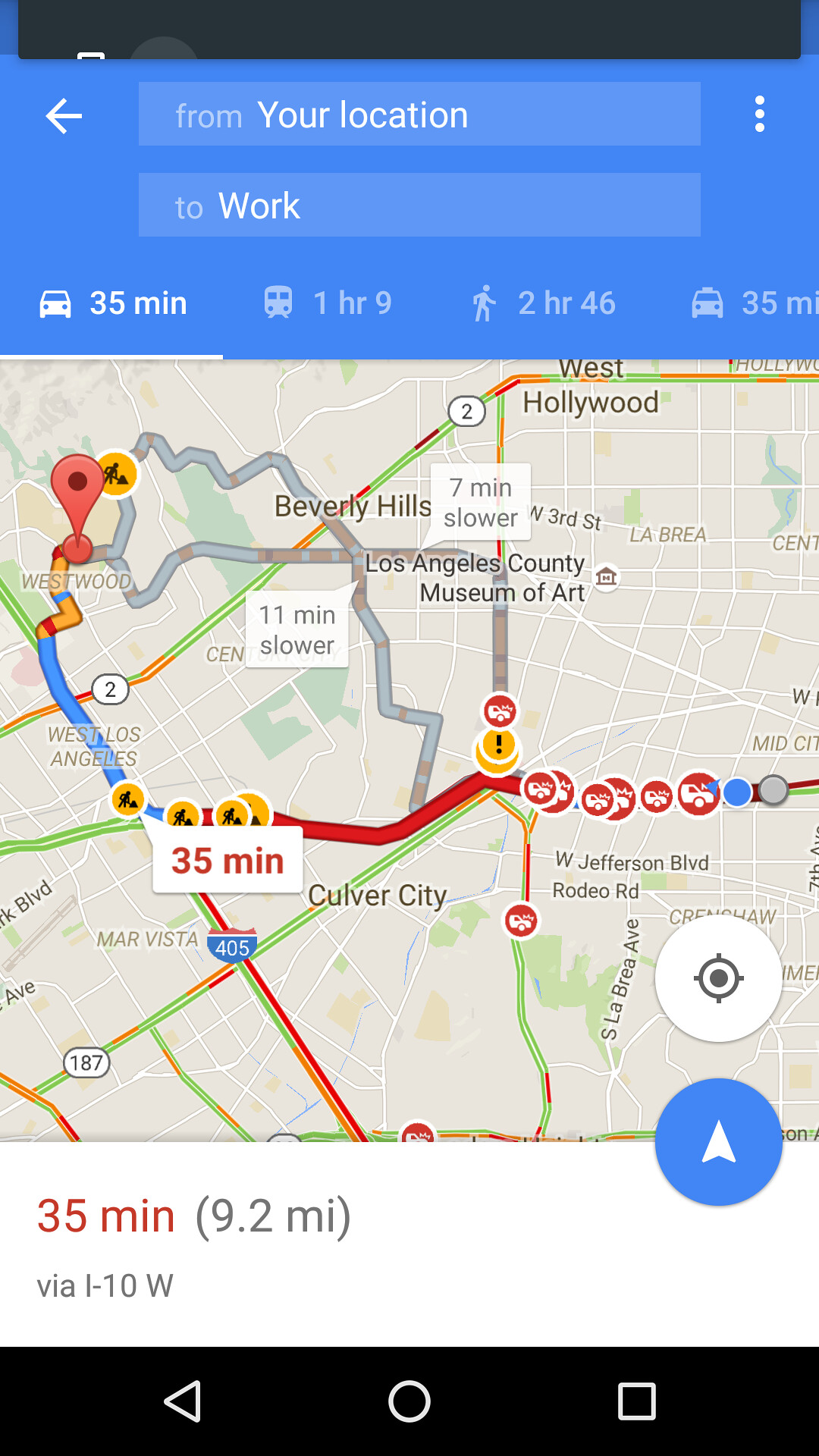This is a detailed color screenshot from a smartphone, displayed in portrait format, which shows a navigational map. The image primarily presents directions from "your location" to "work" using a mapping application similar to Google Maps. At the top of the screen, a blue rectangular bar indicates the starting and ending points of the journey, reporting that it takes 35 minutes to drive.

In addition to the driving time, the screenshot provides estimated travel times for other modes of transportation: 1 hour and 9 minutes by public transit and 2 hours and 46 minutes by walking. The map section below the direction details illustrates the route, showing general street names and red-marked areas indicating heavy traffic. It also highlights several small circles representing car crash sites and includes the primary end destination marked by an arrow.

The bottom of the screen reiterates the driving time of 35 minutes in red, indicating significant traffic congestion, and notes the total distance as 9.2 miles via the I-10 West. These details are displayed above the phone's usual navigation buttons, including a back button, a close button, and additional icons such as a triangle turned to the right, a zero, and a square.